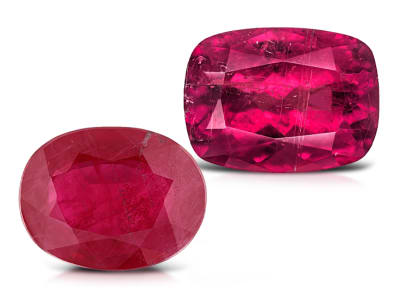The image depicts two meticulously cut, shiny jewels placed against a stark white background. The jewels, which appear to be precious stones, exhibit various shades of red; one is a classic red with a rectangular shape, its sides subtly curved outward, while the other is a reddish-purple oval. Both jewels have black patches scattered across their surfaces, adding to their intricate appearance. Positioned side by side, with the oval jewel slightly below and to the left of the rectangular one, the gems cast distinct shadows underneath each. The overall aesthetic of the image resembles computer-generated clip art, yet captures a photographic quality.